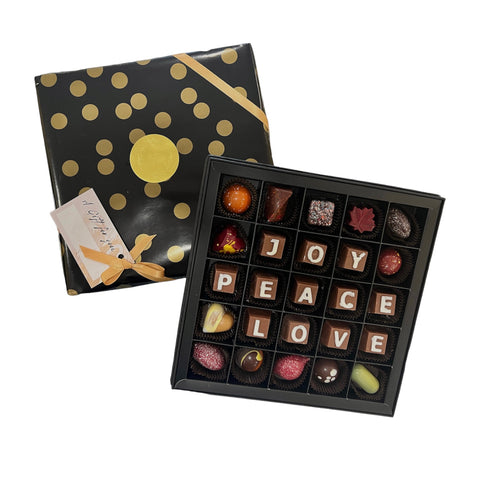This is a detailed photo of an elegantly presented open box of chocolates, with both the lid and the box stood up on their sides to showcase the contents and the decor of the top. The lid is predominantly black, adorned with gold polka dots, and features a black ribbon stripe at the top right corner. Attached to the bottom left of the lid is a gold bow with a card that reads "A Gift For You," leaving space for personalization. The box itself is also black with a checkerboard pattern and contains 25 compartments in a 5 by 5 arrangement. Each square holds a unique, high-end chocolate, except for specific rows that bear inscriptions. The second row has JOY spelled out in white text on brown chocolate squares in the middle three compartments. The middle-most row spells PEACE, and the second from the bottom reads LOVE across four compartments, starting from the second one. The unique chocolates vary in design and color, ranging from a smooth caramel-colored ball, a brown hourglass, a glittery multicolored square, a brown maple leaf, to an obsidian-like piece with black and white speckling. The assortment includes a red and yellow butterfly-like chocolate, a brown sphere, a heart split into yellowish-white and caramel-brown halves, and diverse shapes like an oblong red and white speckled one, a brown sphere with a golden swoosh, a red whoopee cushion shape with white speckles, a jack-o'-lantern-like piece, and a pale matcha-colored piece. These artisanal chocolates appear to be of high quality, ideal for gifting.